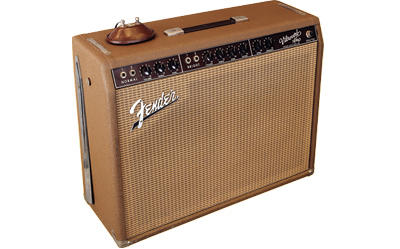This image features a vintage Fender amplifier displayed against a pristine white background, as might be seen on a sales website or at an auction. The amplifier has a distinct light brown housing and a beige and brown front mesh-style speaker cover. Prominently positioned on the upper left corner of the speaker section is the iconic Fender logo, presented in slanted white letters on a black line. Above the logo, a streak of gray runs from the lower back section to the top. The top of the amplifier boasts a variety of knobs, jacks, and dials for tuning and connecting musical equipment, emphasizing its practical and portable design. Additionally, a black handle with silver attachments is affixed to the top, further underscoring its portability.